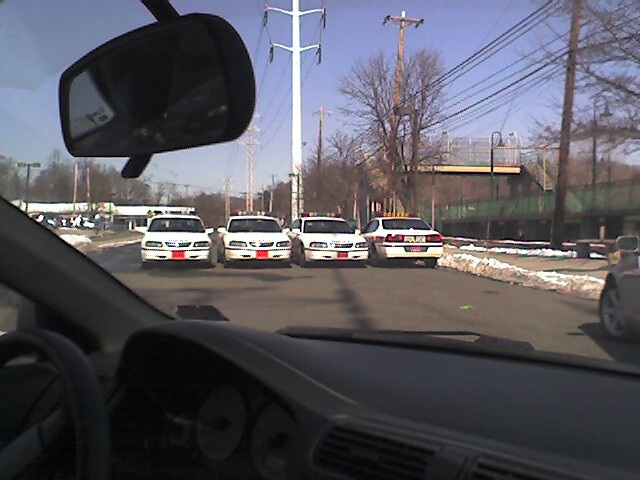This image captures the scene from inside a car, possibly from the passenger seat, with parts of the dashboard, steering wheel, and rearview mirror visible in the shadowed interior. The main focus is on four white police cars, three of which face toward the viewer while the fourth faces away, clearly displaying the word "POLICE" on its back. These appear to be older models with light bars mounted on their roofs. The police cars block the road, likely a highway or street, in an urban setting marked by a high, green, mesh fence that's difficult to see through, several tall bare trees, and numerous utility poles—some wooden, others metallic. Adjacent to the scene is a wide, elevated walkway enclosed in fencing. The blue sky and the remnants of snow on the ground suggest a sunny winter day. Another vehicle encroaches into the frame from the right, showing part of its front wheel and wing mirror. In the distant background, there are hints of a suburban landscape with additional utility poles, possibly a couple of buses, and what appears to be a petrol station toward the far left.